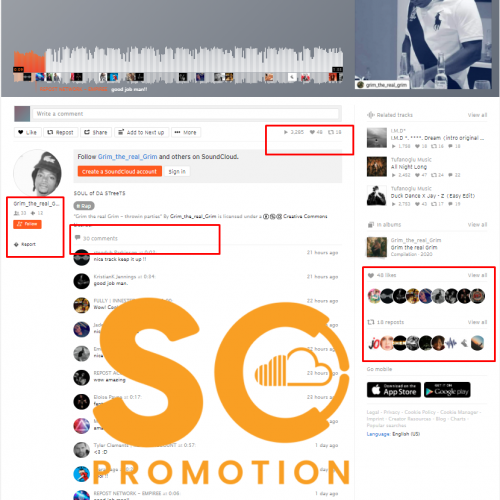This is a screenshot of the SoundCloud app or website, displaying an artist's page with music playing at the top. Several areas of the image have been highlighted with red squares, but the text and imagery within these highlighted sections are too small to discern specific details. Over to the right side of the screen, there appears to be an icon, though it's unclear whether it represents the artist or the user who is logged in. A prominent "SC Promotion" logo is overlaid in the center of the screenshot, featuring the SoundCloud emblem within the "C" of "SC". This suggests the content may relate to a SoundCloud promotion, possibly highlighting an artist that the platform is currently endorsing. Despite the highlights, the text's small size renders the exact purpose and details obscure.